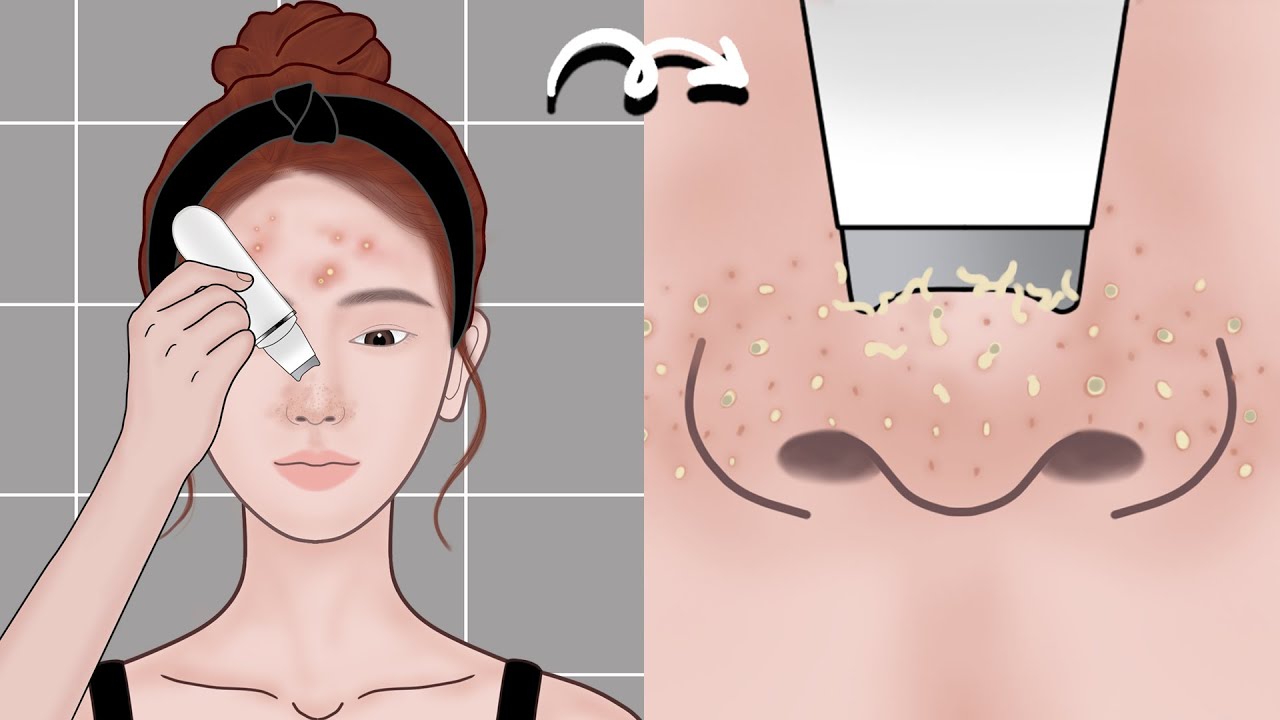The image showcases two detailed, cartoony illustrations positioned side by side. On the left, there is an Asian woman with long, brown auburn hair tied up in a bun, accented by a black headband with a knot on top. She has a black tank top and visible pimples and whiteheads on her forehead and nose. Only her upper body is shown, against a background of grey tiles with white grout lines, resembling a bathroom wall. She holds a white tool designed for pore cleansing, which she uses to scrape her nose.

The right side features a close-up of her nose, demonstrating the tool in action. The white, curved scraper is shown pressing down on her nose, expelling pus and whiteheads from her pores. An arrow with a squiggly line connects the two illustrations, guiding the viewer from the woman to the detailed close-up of the extraction process. The close-up vividly depicts the tool's effect, pushing out yellowish substances from her pores, underscoring the tool's purpose and method of use.